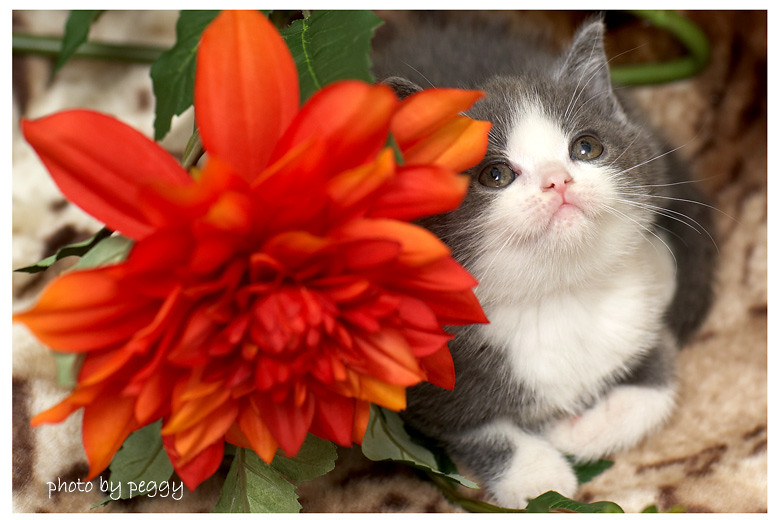A close-up of a young kitten with a gray body and white fur on its face, chest, and paws is resting on a beige and brown rug. The kitten's nose is pink, and it's looking up and away from the camera. Beside it, a large reddish-orange flower with numerous petals and some green leaves is prominently featured. The background includes additional leaves and stems, suggesting it might be taken outside or in an enclosure with plants. The bottom left corner of the image contains a watermark in a fancy font that reads "photo by Peggy."